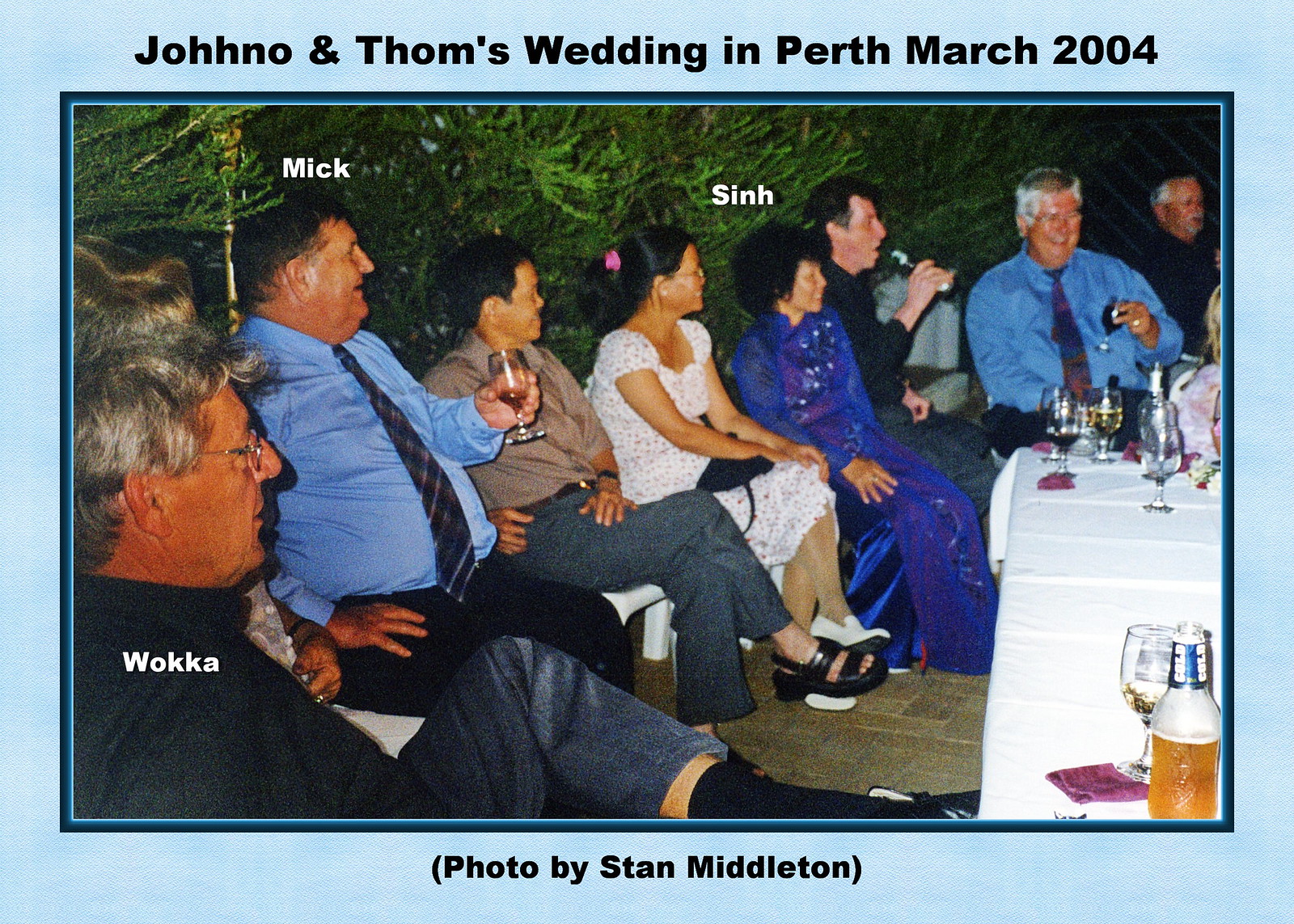The photograph captures a lively moment at Jono and Tom's Wedding in Perth, March 2004. It features a group of nine people, with a tenth person partially visible, all seated in white outdoor chairs around a long white table adorned with a white tablecloth. The table is filled with various drinks, including beers and glasses of wine, and an open bottle can be seen in the bottom right corner. Above the group, in black text, is the caption "Jono and Tom's Wedding in Perth, March 2004," while below the photo, it reads "Photo by Stan Middleton." The setting appears casual yet festive, with everyone dressed lightly, likely due to the warm weather, evident by their jackets being off. The backdrop of bushes hints at an outdoor celebration, contributing to the cheerful atmosphere as guests laugh, smile, and enjoy their drinks together. Some names, like Waka, Mick, and Sin, are written above certain individuals, adding a personal touch to this memorable occasion.